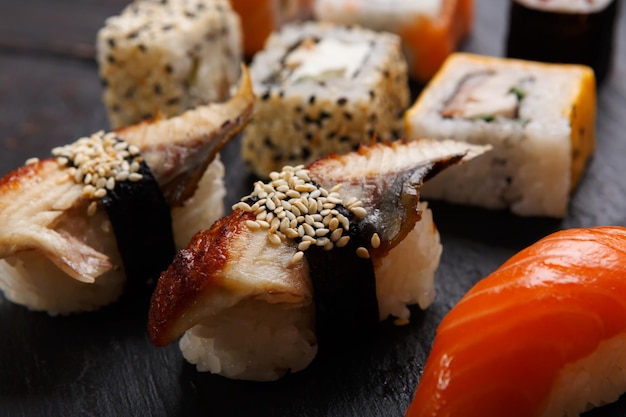The image is a photorealistic, full-color close-up of assorted sushi placed on a dark brown wooden table. In the foreground, there are three individual round pieces of sushi topped with sesame seeds, displaying shades of brown, yellow, white, and orange. Additionally, two distinct pieces of inagi sushi, characterized by their eel topping, are prominently featured. There's also a brightly lit piece of salmon nigiri, with a vivid orange slice of salmon draped over a small ball of rice. In the slightly blurred background, three square-shaped sushi pieces are visible, each encased in rice and sprinkled with sesame seeds. The overall composition is carefully detailed, highlighting the textures and colors of the various sushi pieces against the dark wooden backdrop, with no other objects present.